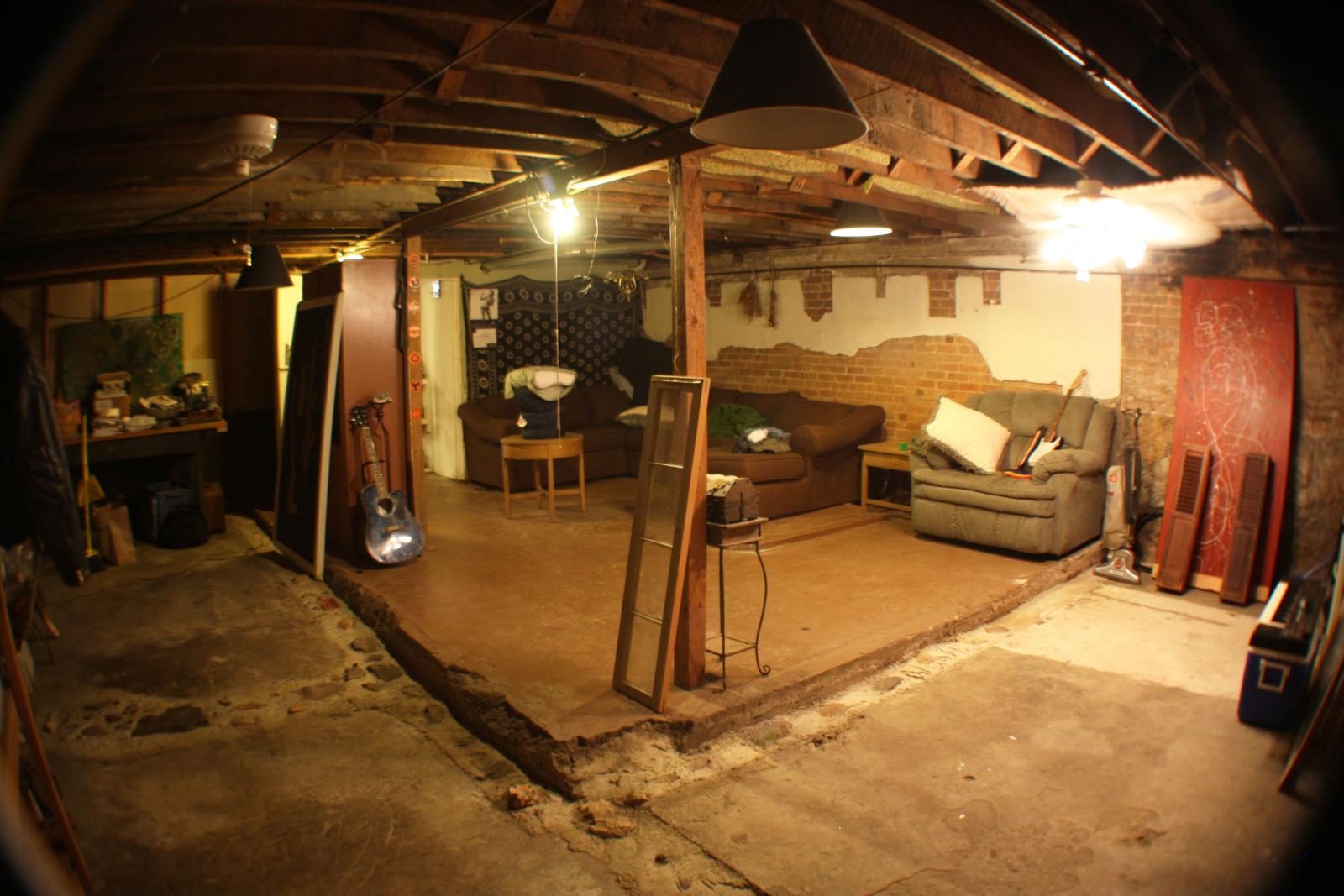The image depicts a rundown basement with exposed wooden beams and bare brick walls, evoking a sense of disrepair. The brown-hued floor is broken and dirty, adding to the neglected atmosphere. Central to the scene is a brightly lit area, with one light hanging from the rafters in the middle of the room and another on the right. Strewn across the basement are various pieces of furniture, including a loveseat, a sofa, and an additional couch. Two guitars are visible: one in the background and another resting on a couch. Among the clutter, a vacuum cleaner leans against the wall near a cooler that has a keyboard placed on top of it. A red poster adorns the right wall, and various small, indistinguishable objects are scattered throughout. A door to a shelf stands in the center, with a toolbox behind it, and a smoke detector is mounted on the ceiling. Despite the general disarray, the scene suggests a semblance of organization amidst the chaos.